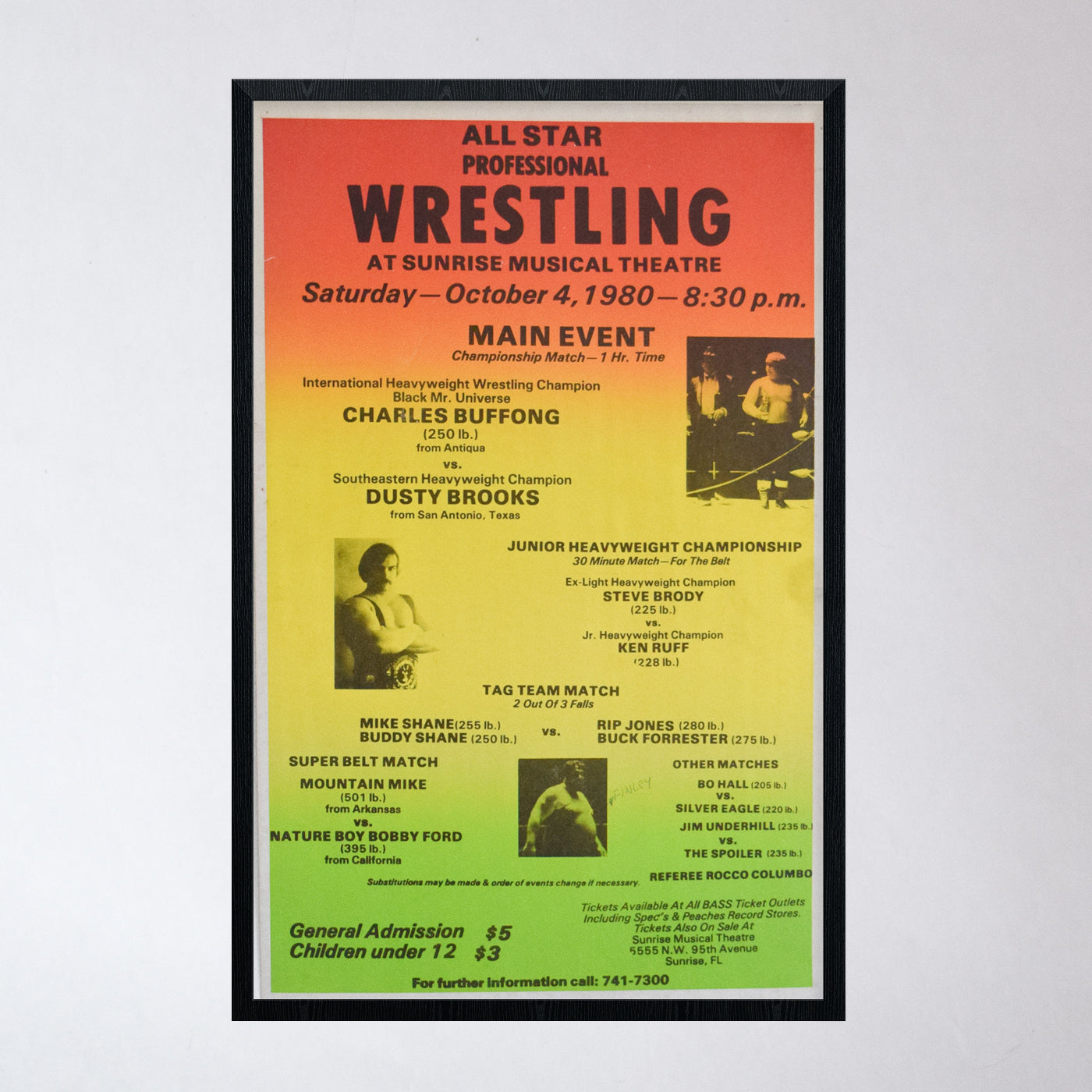This is a vividly colored, framed advertisement for an All-Star Professional Wrestling event held at the Sunrise Musical Theater on Saturday, October 4, 1980, at 8:30 PM. The poster features a gradient background transitioning from red at the top, through yellow in the middle, to green at the bottom, anchored by a bold black border and a white matting. The text highlights key event details in black writing, prominently displaying "All-Star Professional Wrestling" at the top. The main event is a championship match with a one-hour time limit, pitting the International Heavyweight Wrestling Champion, Black Mr. Universe Charles Buffon (250 pounds from Antigua), against the Southeastern Heavyweight Champion, Dusty Brooks from San Antonio, Texas. 

The poster showcases three old-timey photographs: on the top right, a heavyset man standing in a boxing ring; in the middle left, a muscular man wearing a trophy belt; and at the bottom center, a particularly overweight man. Further event details include a match between Steve Brody and Ken Ruff, the Shane Brothers vs. Rip Jones and Buck Forrester in a tag team match, a super belt match featuring Mountain Mike vs. Nature Boy Buddy Ford, and additional bouts such as Bo Hall vs. Silver Eagle and Jim Underhill vs. The Spoiler. Ticket prices are listed as $5 for general admission and $3 for children under 12, with a contact number for further information.